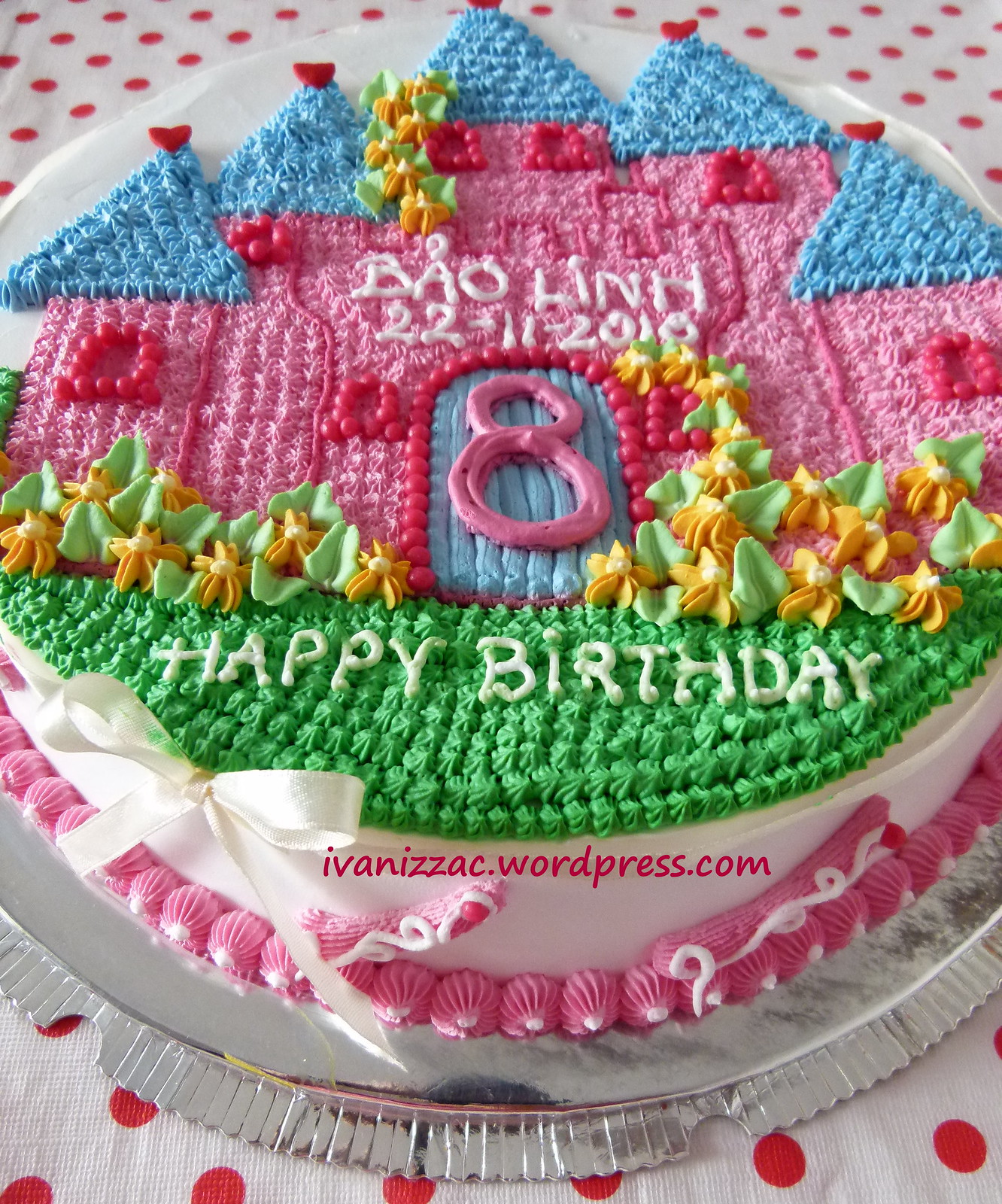This vibrant and colorful children's birthday cake features a stunning single-layer design, primarily frosted in white. Dominating the top is a meticulously crafted pink castle, embellished with blue turrets capped with red flag-like peaks. The castle boasts red windows and a prominent blue door adorned with the number 8 in pink frosting. Above the door, in white icing, are the words "Bao Lin, 22-11-2010," though the date could also be "22-11-2016." The cake is further decorated with yellow and green floral details and green icing at the base, simulating grass. The cheerful message "Happy Birthday" is also inscribed in white frosting on the green base. Completing the design, a dark pink border with white dots edges the bottom of the cake, which is wrapped in a white ribbon. The cake sits on a translucent plate atop a white tablecloth with red polka dots. Superimposed on the photograph is the text "ivannezac.wordpress.com."